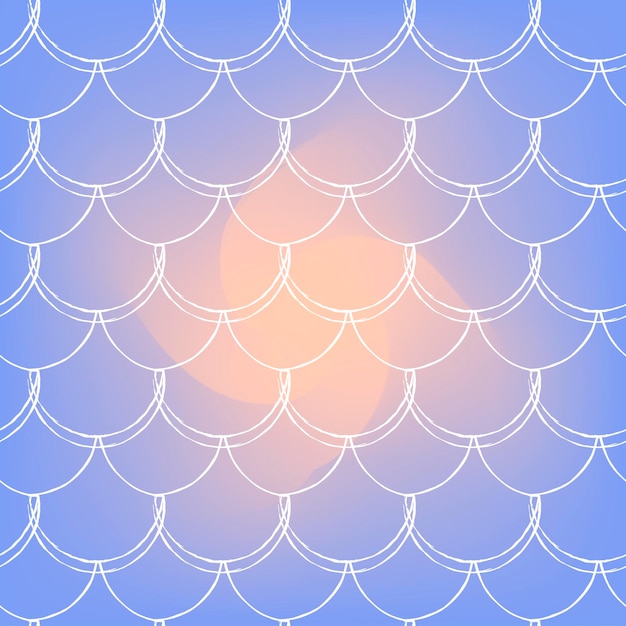The image is a simplified, computer-generated drawing featuring a central, tan to light orange quad swirl, resembling a four-lobed pinwheel that appears to turn counterclockwise. Surrounding the central swirl is a light blue background. Overlaying the entire image, including the swirl, is a uniform pattern of thin, semi-circular white lines that intertwine and repeat, creating an effect reminiscent of fish scales or chain mail. These white lines, likely drawn with a virtual marker, span the entire image, adding a textured layer that merges with both the tan pinwheel and the blue backdrop.